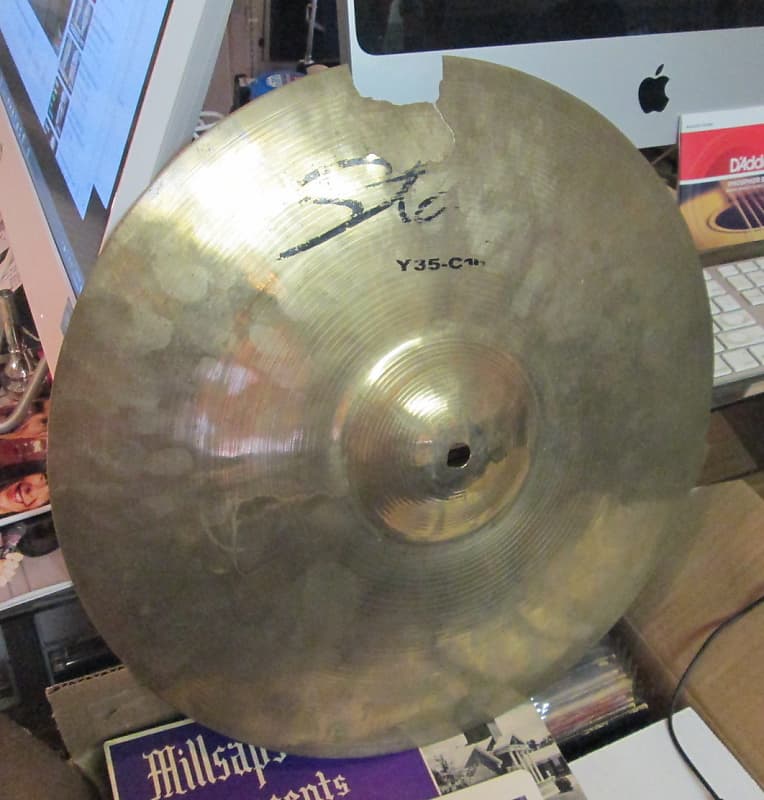This image showcases a large, shiny brass cymbal, heavily dominating the scene. The cymbal, typically part of a drum set, is positioned upright against a wooden box, facing the viewer, and exhibits a prominent crack near its top. It's adorned with black, faded lettering, partially revealing "STA" in a curly font and a clearer "Y35-C". Below the cymbal, there's an object that appears to be sheet music or possibly an album cover, partially obscured with indistinct text that may read "Millsaps". In the background, two Apple computers are visible; the one on the left is turned on, displaying a webpage, while the other on the right, along with a white Apple keyboard, is turned off. Adjacent to the computers are several framed pictures, their contents mostly out of frame and indiscernible. The entire composition suggests a workspace, with the cymbal perhaps placed for examination.